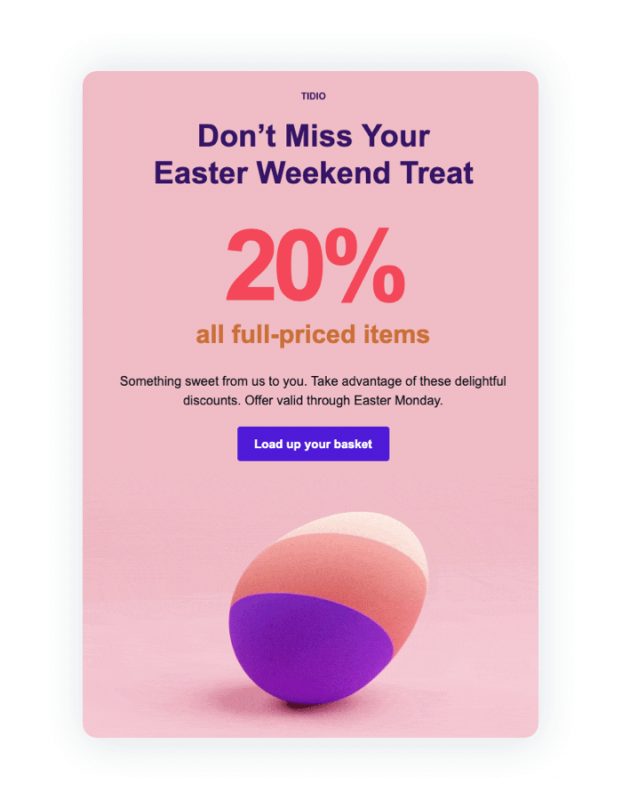**Advertisement Caption:**

This vertical rectangular advertisement sits on a light pink background. At the top, in very small, all-capital, purple font, it reads "TIDIO". Just below that, in a larger purple font with only the first letter of each word capitalized, it states "Don’t Miss Your Easter Weekend Treat."

Further down, in a coral color, the ad displays "20%". Below, in a golden-yellow orange color, the text reads "all full-priced items," entirely in lowercase.

In small black font under that, it offers a short message: "Something sweet from us to you. Take advantage of these delightful discounts, offer valid through Easter Monday."

A bright purple horizontal rectangular box follows, with bold white font that prompts, "Load Up Your Basket."

At the bottom of the image, there is an Easter egg illustration divided into three horizontal sections by color. The top third is white, the middle third is coral, and the bottom third is bright purple. The egg is lying on its side with the pointed white section facing the upper right corner, while the bottom rests slightly left of center.